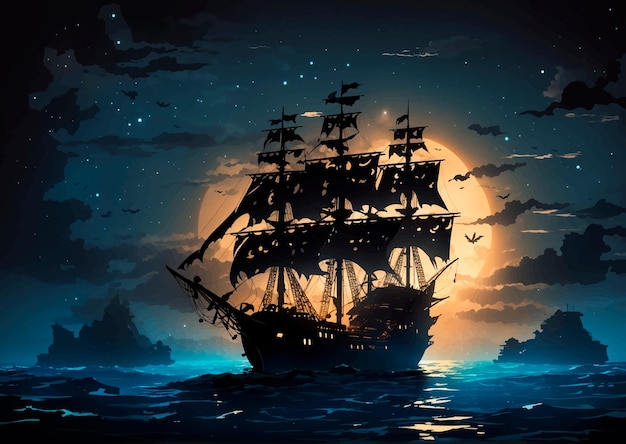The image depicts a detailed anime-style digital drawing set during nighttime. The sky, a deep navy and midnight blue, is dotted with white stars and sporadic dark clouds. In the backdrop, a large, glowing orange moon provides a dramatic contrast. Centered in the composition is a considerable pirate ship, characterized by its tall, layered masts and black sails, all marred with holes and tears, signaling damage. The ship's dark silhouette stands out against the ocean's dynamic interplay of blue and white waves. In the background, there are vaguely visible landmasses on either side, and a few birds are captured in flight, adding to the sense of a vast, tumultuous seascape. The overall image is vibrant and clear, with excellent use of color and lighting to enhance the nocturnal, slightly eerie atmosphere.